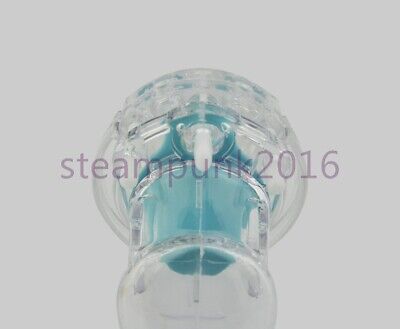Set against a light gray background, this square image prominently features the text "Steampunk 2016" across its middle. Captured from the viewpoint of someone beneath the object, the photograph showcases a glass structure resembling a stemmed glass with a rounded base, cylindrical stem, and a cup-like top. Inside this glass object, there is a distinctive green candle with a face-like shape looking down into the camera. The candle's green hue contrasts with the dark green details of the face, including green eyeballs. Above the candle, the glass cap has an intricate green trim, giving a steampunk aesthetic to the overall image. The setting appears to be indoors, adding to the photographic realism of the composition.